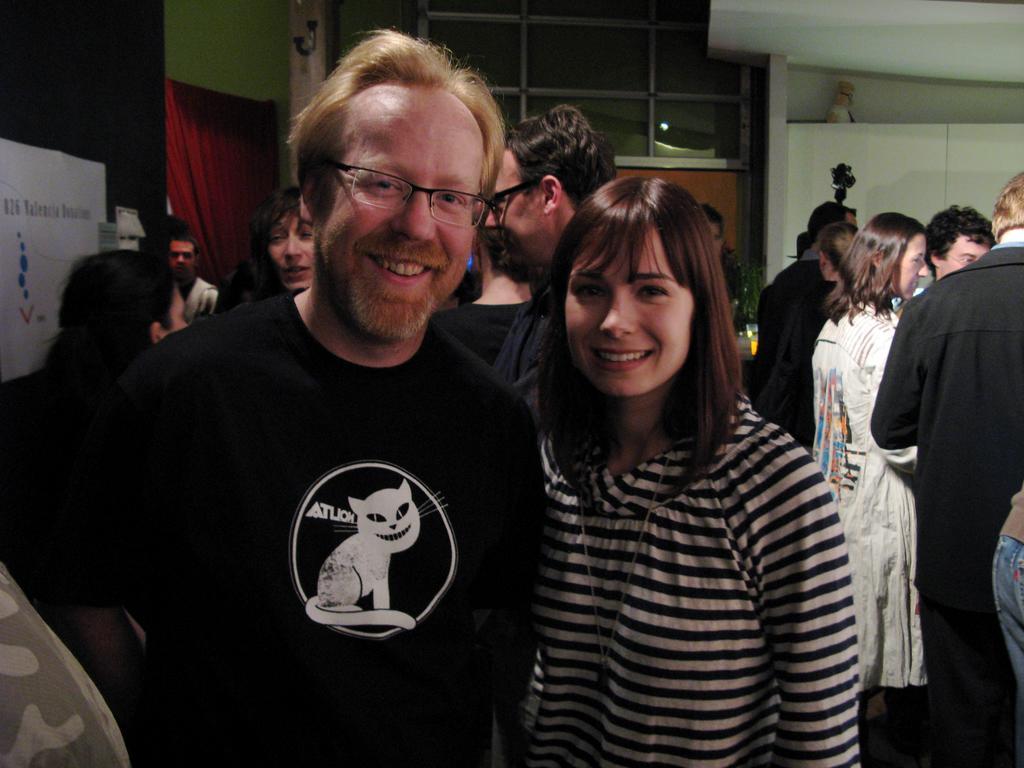In the center-left of this photo from a casual event among friends, the focal point is a smiling gentleman and a woman beside him. The gentleman on the left is easily identifiable by his black, top-rimmed glasses with clear bottoms. He has thin, reddish hair that is slightly receding and neatly cut. His slightly graying beard and reddish mustache add to his distinguished look. He is wearing a black t-shirt featuring a quirky design: a white caricature of a cat with a swirling tail and slanting black eyes, giving off a devilish grin, all set within a circular motif. To his right stands a woman who appears to be in her early to mid-thirties, slightly younger than the man who seems to be in his forties. She has a cheerful expression and is dressed in a stylish black blouse with alternating black and white stripes of equal width, and a ruffled collar that adds a touch of elegance. Her brunette hair frames her face nicely as she smiles for the camera. In the background, people can be seen milling around, adding to the lively, convivial atmosphere of the event.